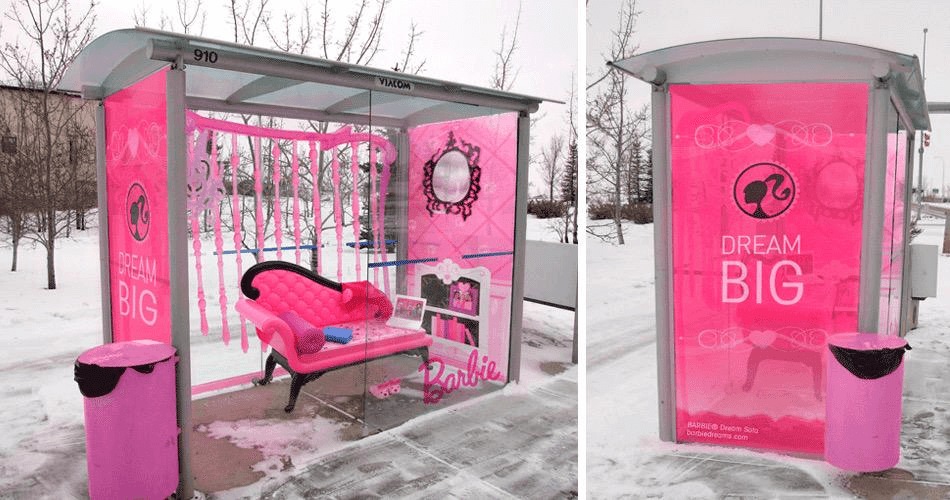The image captures a snowy, winter scene of a stylish Barbie-themed bus stop under a dark gray, heavily clouded sky. The ground is covered with heavy snow, and surrounding the bus stop are leafless, brown trees. The bus stop itself features a sleek, gray metal frame with a partially transparent, shaded roof. Its base is made of gray concrete. A distinct pink trash can stands to the left, with a black trash bag inside.

The bus stop’s interior is uniquely decorated to resemble a cozy, vintage room. It houses a single, luxurious pink reclining settee with a quilted upholstery back and dark wooden legs, ornamented with a pink neck roll. Artful details include painted pink panels and a mirror with a black ornate frame inside, enhancing the chic aesthetic. The left side of the bus stop displays a pink poster reading "Dream Big," featuring a black silhouette of Barbie's head and ponytail. The front glass has "Barbie" elegantly painted in pink. The right side of the bus stop continues the theme with a matching pink wall application bearing the Barbie logo, while a white painted shelf with pink books adds to the whimsical decor.

The image is presented as two black-and-white photographs side-by-side, with the left side showing a wider landscape view and the right side focusing on a close-up of the "Dream Big" text and Barbie silhouette. These combined photographic and illustrative techniques give the overall scene a surreal yet detailed realism, blending representational imagery with creative embellishments.